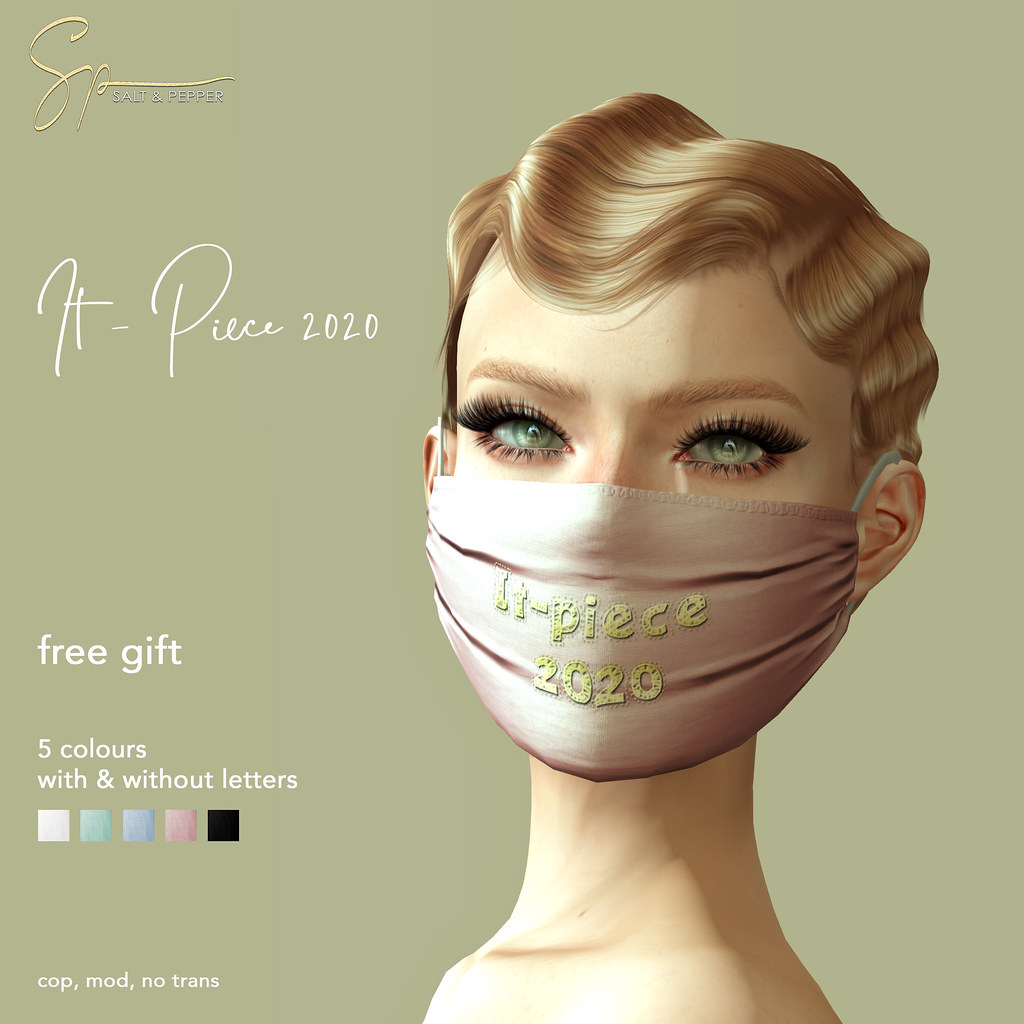The image appears to be an advertisement featuring a possibly AI-generated woman centrally positioned with a distinct, stylized look. She has long, black eyelashes and light brown or blonde hair. The woman is wearing a pale pink mask that says "ITPEACE 2020," which hooks over her ears. Her skin is light brown. The background of the image is a yellowish-green hue, and the text appears in white. "Salt and Pepper" (SP) is likely the brand being advertised, as indicated by the logo. The advertisement mentions a free gift available in five colors, with or without letters: white, green, blue, pink, and black. The text is positioned on the left side of the image, emphasizing the offer and the brand. Overall, the ad promotes stylish, customizable masks through a visually striking and modern design.